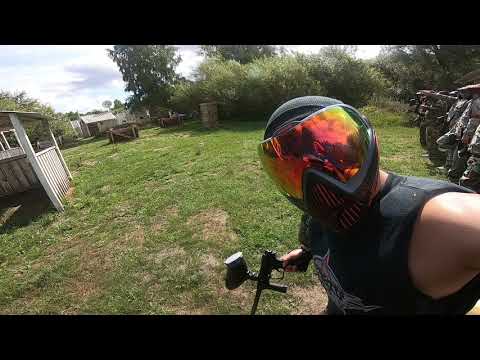A full-color landscape photograph taken outdoors during a partly cloudy day shows a person taking a selfie in the bottom right corner. The image features a black border on the top and bottom. The person, wearing a black tank top with a white graphic and a helmet with a multicolored reflective visor, is gripping a paintball gun, not a motorbike handle as initially thought. They appear to be in a grassy yard, possibly their backyard, surrounded by several old wooden buildings and outbuildings to the left, with trees and bushes framing the scene to the right. In the far left background, there are what appear to be rocks and a structure resembling a ramp. The overall aesthetic of the photograph is representational and realistic.